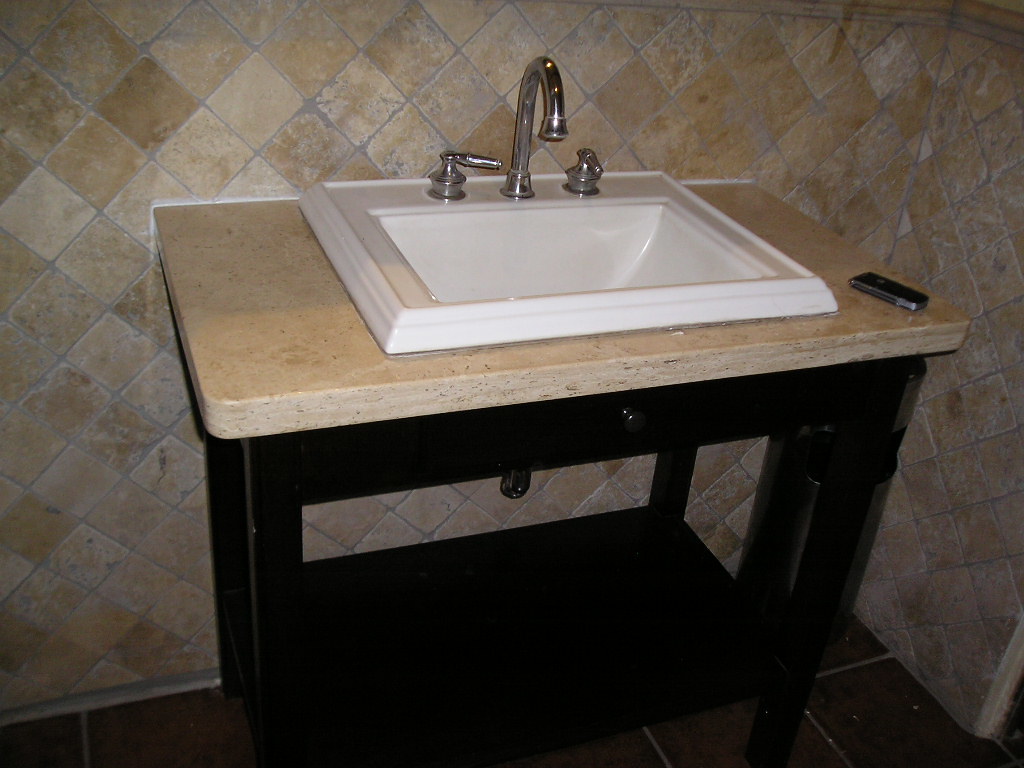This photograph, taken in a bathroom, showcases a horizontally-oriented kitchen vanity. The floor is covered with dark brown tiles, while the wall tiles present an aesthetically pleasing mix of earth tones including yellows, oranges, and browns. These wall tiles are arranged in a diamond pattern, where square tiles are positioned with their vertices pointing up, down, left, and right.

The vanity features a piece of marble, which extends from the wall and shares a similar color palette with the surrounding tiles. Atop the marble is a sleek raised sink, rectangular in shape but appearing trapezoidal when viewed at sink level. The sink is complemented by a modern faucet accompanied by two coordinating knobs.

On the lower right-hand side of the counter, there is an electronic device, although its exact function is unclear. The vanity itself is designed with an open layout; a drawer is visible beneath the counter, encompassed by a black wood frame. The open structure underneath the sink allows for additional storage, possibly for towels or other bathroom essentials, with the backdrop of wall tiles adding a cohesive visual element.

The lighting in the image is dim, creating shadows that grow more pronounced toward the lower part of the vanity, adding to the photograph's moody ambiance.